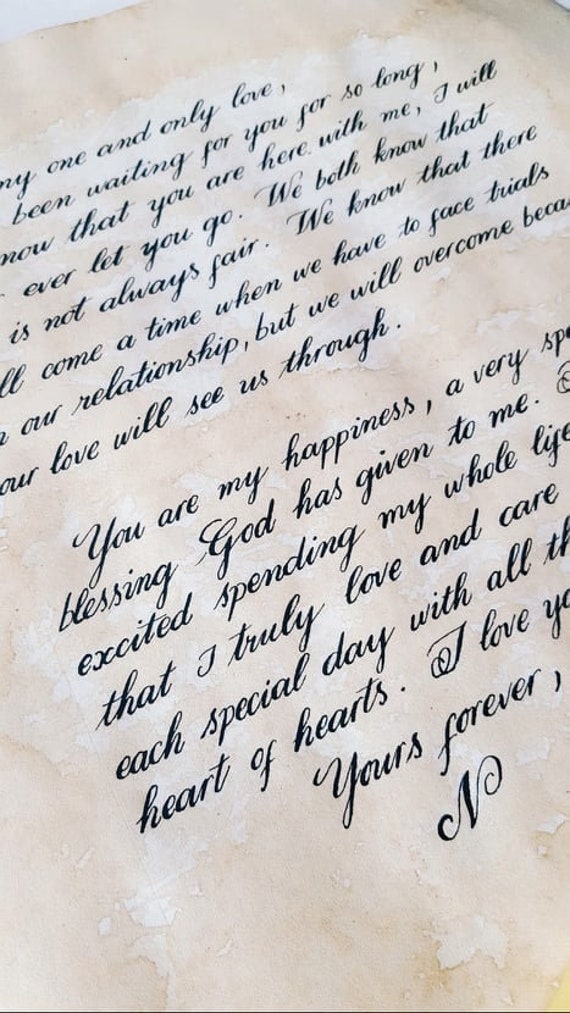The image depicts a slightly angled photograph of an old, beautifully handwritten love letter on weathered beige parchment, possibly resembling paper from 200-300 years ago. The letter, written in elegant, script-like cursive, begins with "My one and only love" and is signed off with "Yours forever, N." The text, partially obscured and cut off at both the left and right edges due to the diagonal angle of the photograph, expresses a deep, undying love. It mentions the anticipation of being together, a promise never to let go, and an acknowledgment of the trials they may face in their relationship. Despite these challenges, the writer is confident that their love will see them through, declaring, "You are my happiness, a very special blessing God has given to me." The letter conveys excitement about spending their life together, cherishing each special day with all their heart.